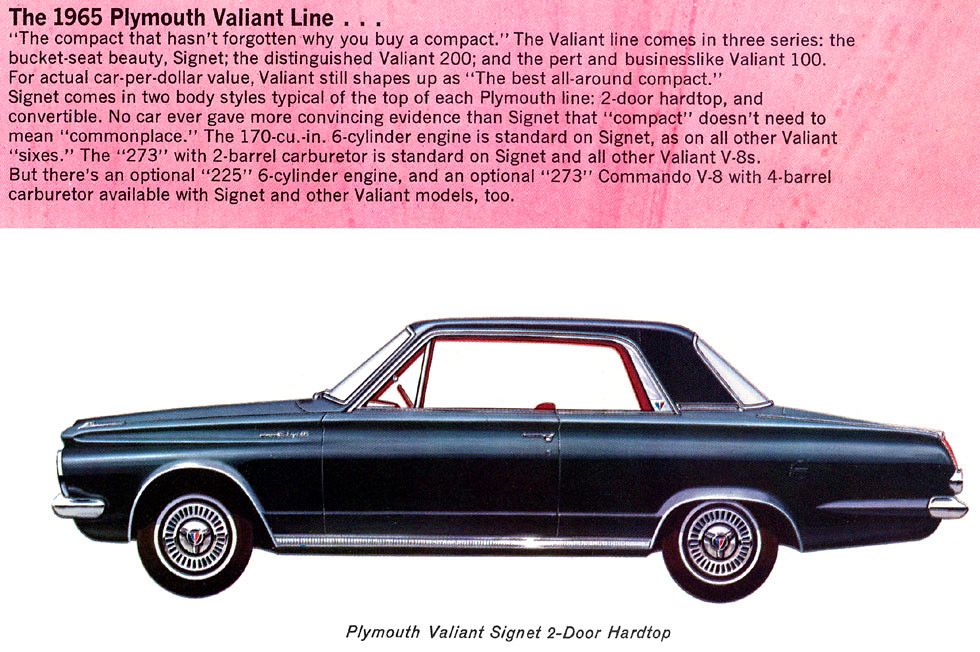The illustration showcases a black, 1965 Plymouth Valiant Signet Two-Door Hardtop, featuring the classic elongated design and silver hubcaps typical of the era. The car is depicted without a B-pillar, emphasizing its hardtop style, and features distinctive silver bumpers. Above the car, a large pink rectangular banner with left-aligned black text reads: "The 1965 Plymouth Valiant line: The compact that hasn't forgotten why you buy a compact." This banner details the three series within the Valiant line: the "Bucket Seat Beauty" Signet, the "Distinguished" Valiant 200, and the "Pert and Business-like" Valiant 100. It also elaborates on the car's specifications, mentioning the standard 175 cubic inch six-cylinder engine and available optional engines, including a 225 six-cylinder and a 273 cubic inch Commando V8 with a four-barrel carburetor. The Signet model is noted for its two available body styles—two-door hardtop and convertible—showcasing that compacts need not be commonplace, but can offer exceptional value and performance.